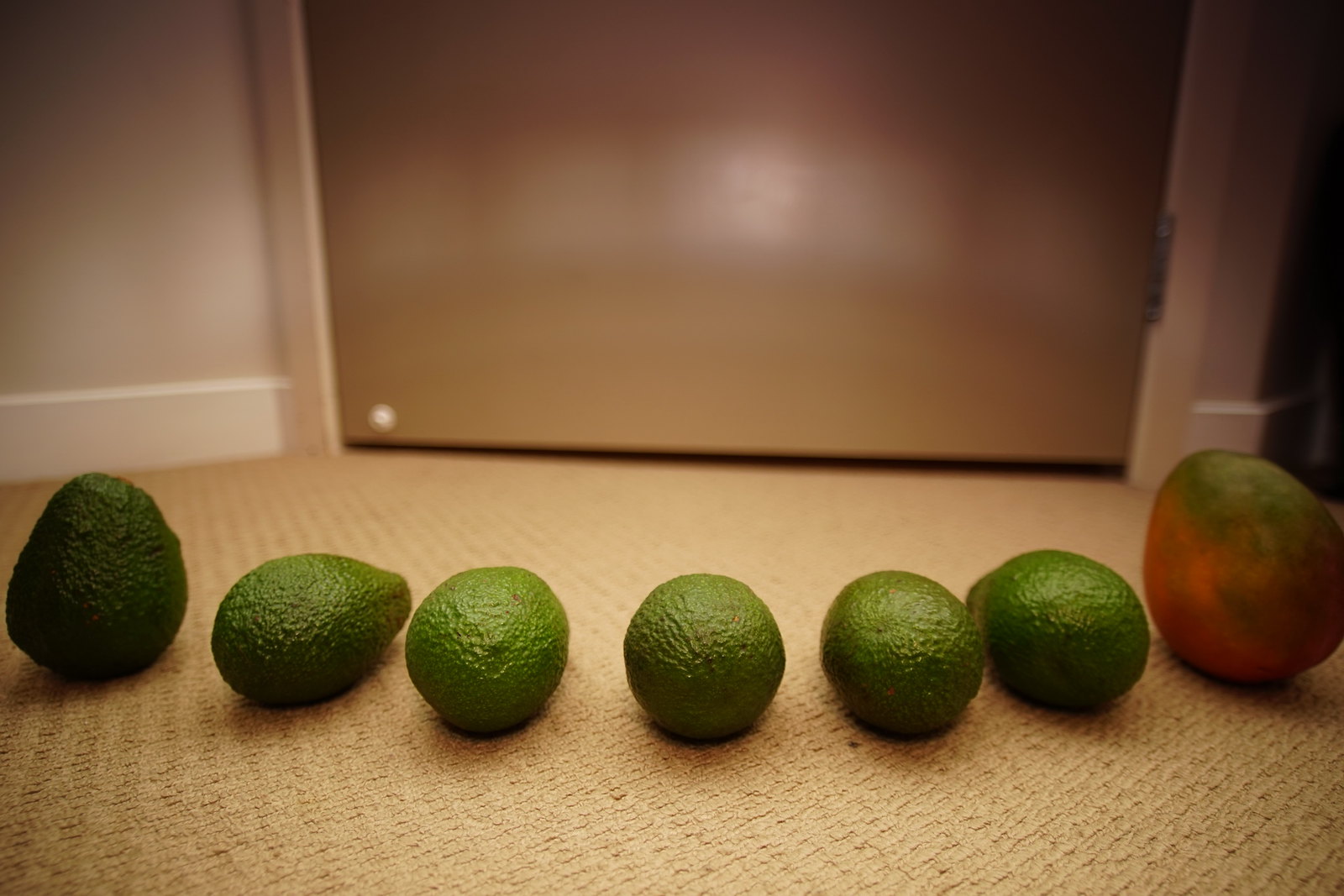In this photograph taken indoors, seven avocados are lined up on a wheat-colored, slightly rough carpet, which evokes the type commonly seen in hotels. The avocados are arranged from left to right, with six of them being green Haas avocados and the one on the far right being green with a rosy-red tint, likely a papaya rather than an avocado. The five middle avocados are positioned with their pointed ends facing away, while the avocado on the far left stands upright on its broader end. The backdrop features a bronze-colored door with a strip of black visible underneath it, framed by white molding and creamy-colored walls, giving the scene a somewhat modern-art feel. The lighting is soft and light, highlighting the texture of both the avocados and the carpet.